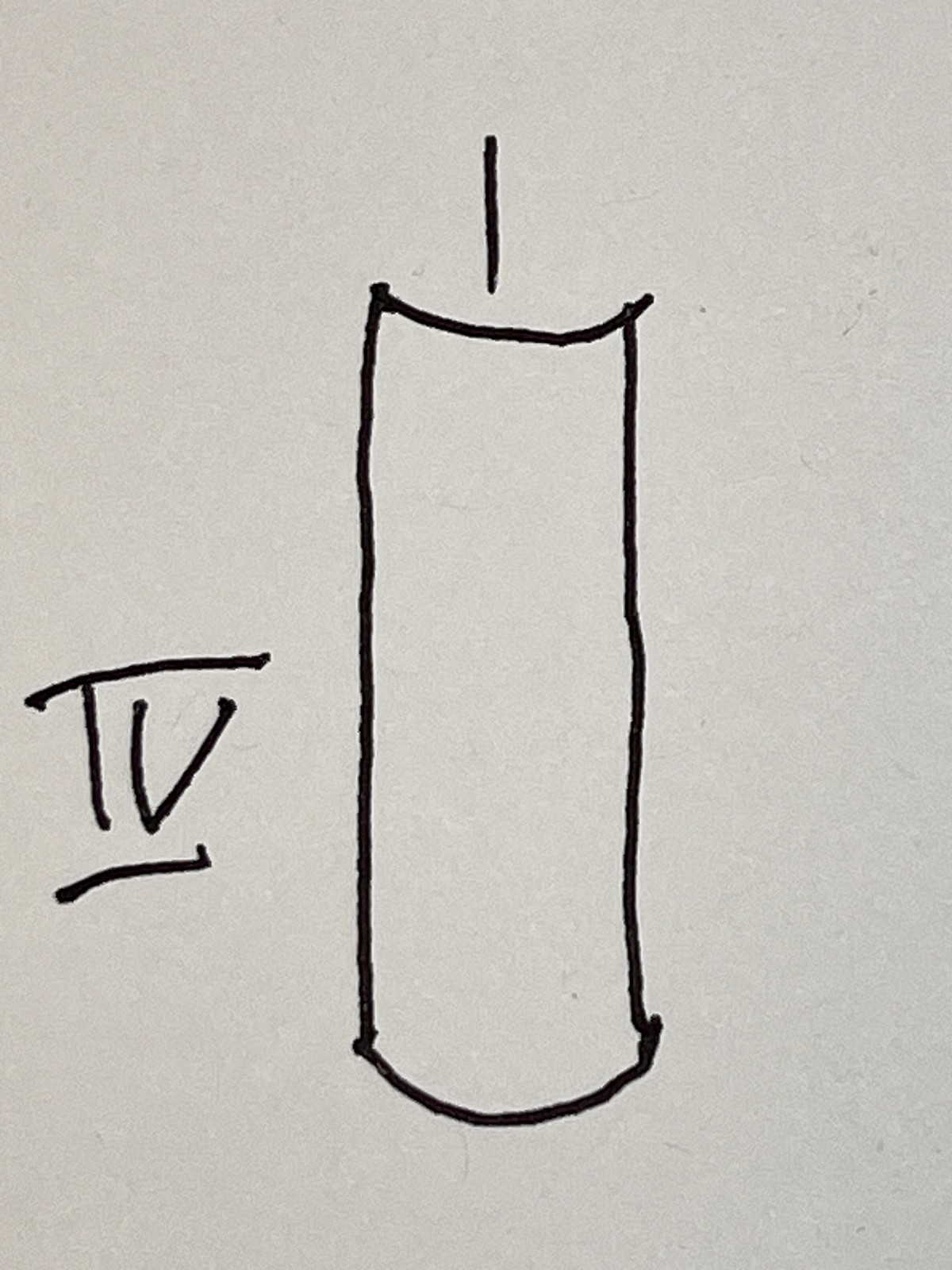This image depicts a minimalist and rudimentary black pen drawing on slightly discolored, off-white paper. The paper exhibits slight gray discoloration in its corners, likely due to age or handling. In the top left corner, the number four is represented in Roman numerals ("IV"), drawn with precise, thick black lines forming a horizontal bar at the top and bottom, a vertical line, and a "V".

Central to the composition is a simplistic depiction of a pillar candle. The candle is represented through basic geometric shapes: a prominent, thick black line symbolizes the flame, rising upwards from the candle. Below the flame, a semicircle at the front forms the top portion of the candle, while two vertical lines extend downward, suggesting the candle's height. The drawing deliberately omits a full circular top, opting instead for a partial representation that emphasizes the candle's front view. The overall art style leans towards abstract minimalism, with thick, confident line work contributing to its stark and striking visual impression.